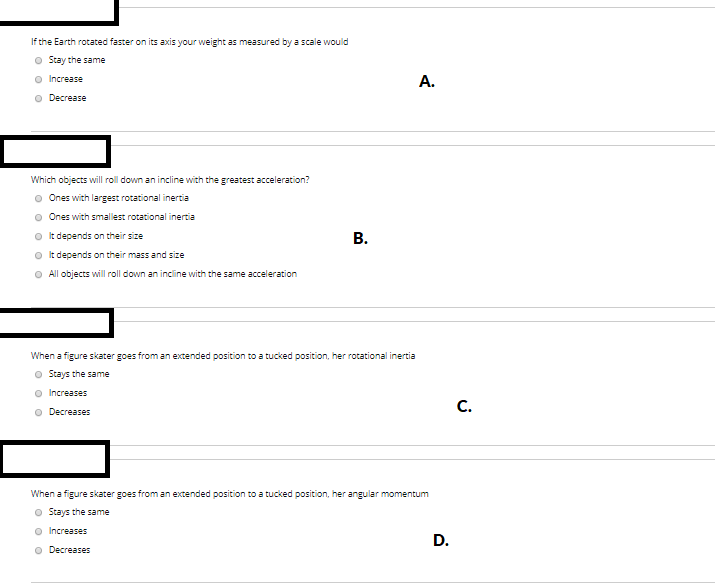The image features a set of four white blocks, each with a distinct black square located in the upper left-hand corner. In the center of each block, there is a different letter displayed prominently in bold.

1. **Block A**: This block prominently features a bold letter 'A' in the center, followed by a period. The block contains a prompt that reads, "If the Earth rotated faster on its axis, your weight as measured by a scale would:" Below this prompt is a multiple-choice question with three possible answers: 
   - Stay the same.
   - Increase.
   - Decrease.

2. **Block B**: This block prominently features a bold letter 'B' in the center. It presents a question and multiple-choice options related to physics, specifically about rolling objects and inertia. The question is: "Which objects will roll down an incline with the greatest acceleration?" The answer choices provided are:
   - The ones with the largest rotational inertia.
   - The ones with the smallest rotational inertia.
   - It depends on their size.
   - It depends on their mass and size.
   - Objects will roll down an incline with the same acceleration.

The remaining two blocks (C and D) are not described in the provided text, and therefore, it is assumed that only blocks A and B are detailed for this image.